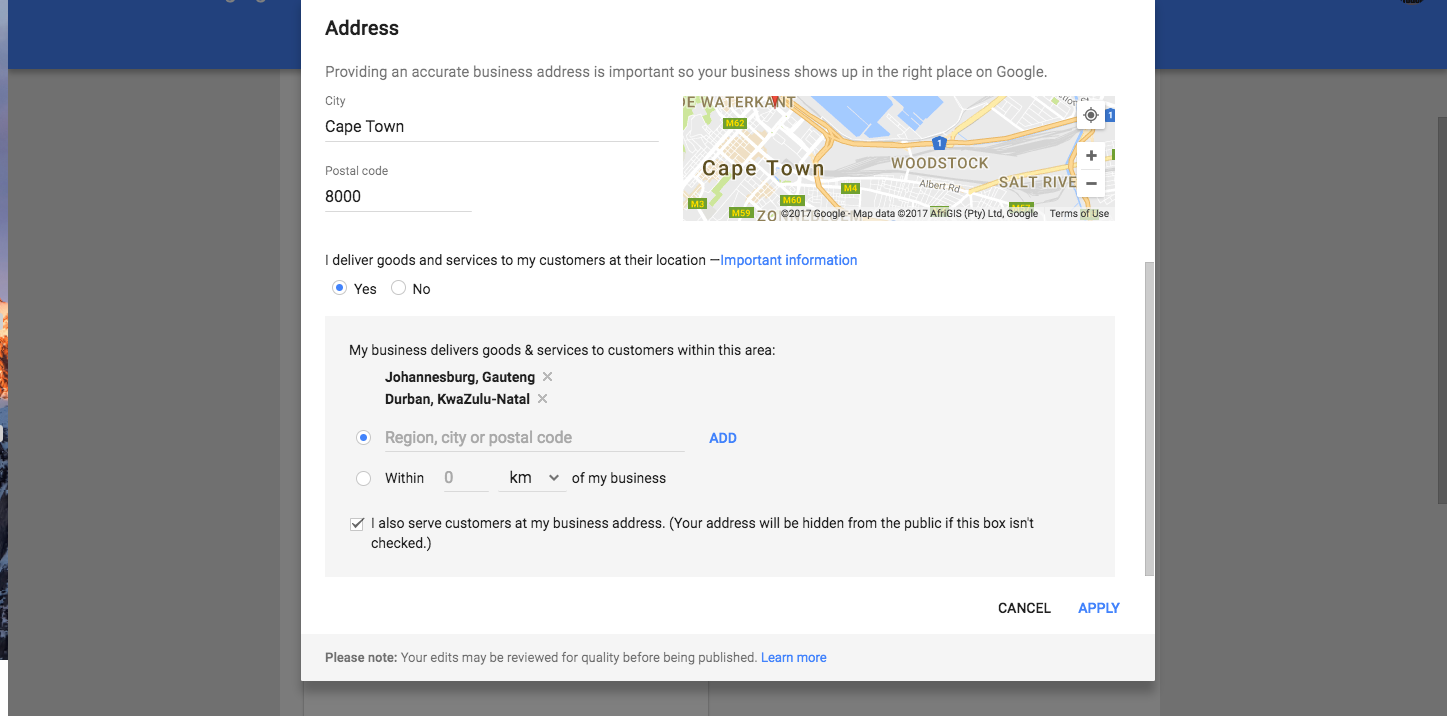**Detailed Google Maps Business Addition Screenshot Description:**

The image portrays a user's desktop interface, featuring a Google Maps business setup screen with a gray background. Dominating the screen is a prominent white rectangular overlay where the business address information is to be entered. At the top of this overlay, a heading labeled "Address" prompts the user to provide their business location. A subheading emphasizes the importance of inputting an accurate business address to ensure proper placement on Google Maps.

Beneath the heading, the fields for "City" and "Postal Code" are filled in with "Cape Town" and "8000," respectively. Below these fields, a wide, but not overly tall, map of Cape Town is displayed, providing a visual reference for the location.

Towards the bottom of the form, there is a question asking whether the business delivers goods and services to customers at their locations with a pre-selected "Yes" option. This section further expands to indicate that the business serves customers within several regions: Johannesburg (Gauteng), and Durban (KwaZulu-Natal).

Additional options appear below, including radio buttons letting the user specify their service area either by "Region, city, or postal code" (selected by default) or "Within a certain number of kilometers of my business."

There is also a checkbox option labeled "I also serve customers at my business address." A note informs users that if this box is unchecked, their business address will be hidden from the public.

At the bottom of the overlay, there are three buttons: "Cancel," "Apply," and a disclaimer stating, "Please note, your edits may be reviewed for quality before being published."

In summary, the image provides a comprehensive view of the steps required to add a business to Google Maps, emphasizing the importance of accuracy and the options available for specifying service areas and customer interactions.